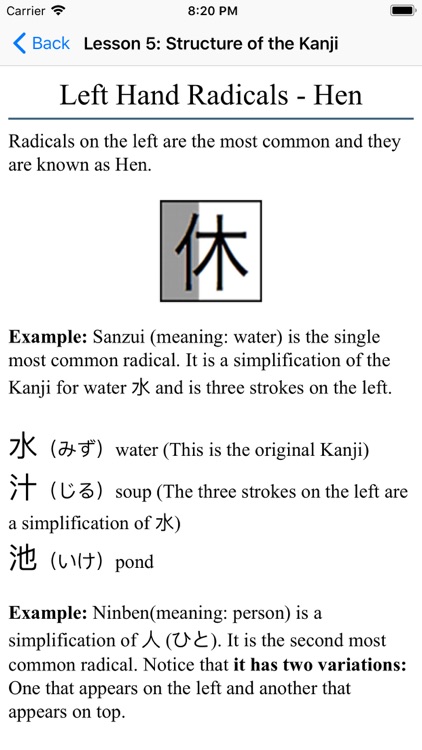The image is a black-and-white screenshot from an educational app on a smartphone, teaching Japanese Kanji. At the top, the interface displays "Lesson 5, Structure of Kanji." A navigation bar features a blue "Back" button in the upper left corner, confirming it is a smartphone app as indicated by the carrier signal, Wi-Fi symbol, and battery status in the top corners, with the time shown as 8:20 PM.

The lesson title reads "Left Hand Radicals - Hen," with a description explaining that "Radicals on the left are the most common, and they are known as Hen." Below the title, an image of a Kanji symbol is displayed, illustrating the radical. The text further explicates the simplification process of these radicals. An example provided is "sanzui," meaning water, identified as the most common radical, consisting of three strokes on the left side of the Kanji for water. Another example, "ninben," meaning person, is also detailed as the second most common radical, offering insight into its variations in placement within characters.